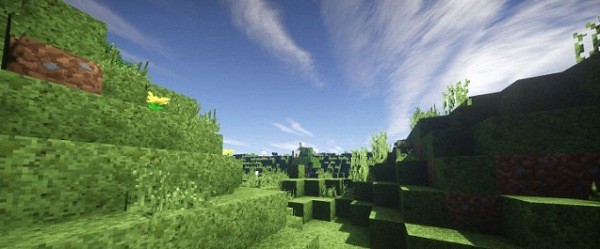The image depicts a computer-simulated hilly landscape reminiscent of the game Minecraft, characterized by its stepped terrain composed entirely of green blocks. The hill features tiered levels, appearing as if one could climb them like stairs. Scattered across the green blocks are patches of trees, weeds, and grass, with notable details including a single yellow flower and a brown patterned block on the side of the hill. The sky above is a clear blue adorned with long bands of wispy white clouds. Although primarily green and blue, the scene also includes small, distinct touches of yellow and brown, adding to the detailed, blocky texture of the environment. The right side of the image is cast in heavy shadow, further emphasizing the depth and dimensionality of the blocky landscape.